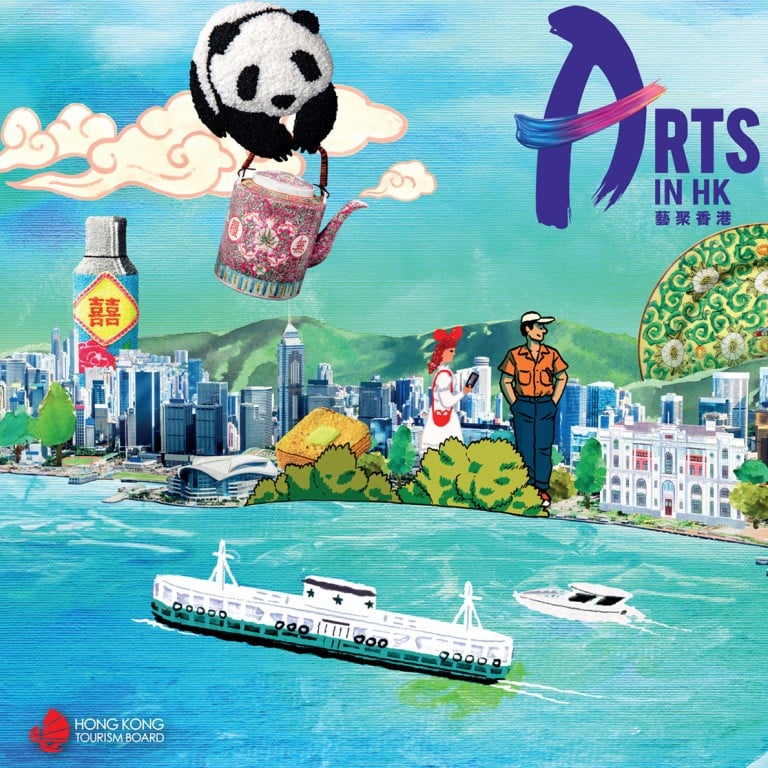This vibrant and surreal Hong Kong tourism board poster, rendered in a colorful cartoon style, prominently features the text "Arts in Hong Kong" in purple letters at the upper right corner. The bustling cityscape along a picturesque river is depicted with a unique blend of realism and whimsy. Two towering Caucasian tourists—a woman in a white dress and red hat, and a man in a yellow shirt with blue pants—stand imposingly among the skyscrapers, emphasizing their vibrant presence. The leftmost building carries a vertical ad extending from the ground to its peak. Below, two boats navigate the water: a lengthy ship and a smaller boat trailing behind. Intricately detailed, the scene also includes lush greenery, various constructions, a bottle featuring Chinese caricatures, and an assortment of local food items scattered throughout the city. Dominating the sky is a fantastical image of a flying panda bear holding a pink watering can, adding a touch of surreal charm to the overall composition. The bottom of the poster reads "Hong Kong Tourism Board," tying together the creative and inviting depiction of Hong Kong.